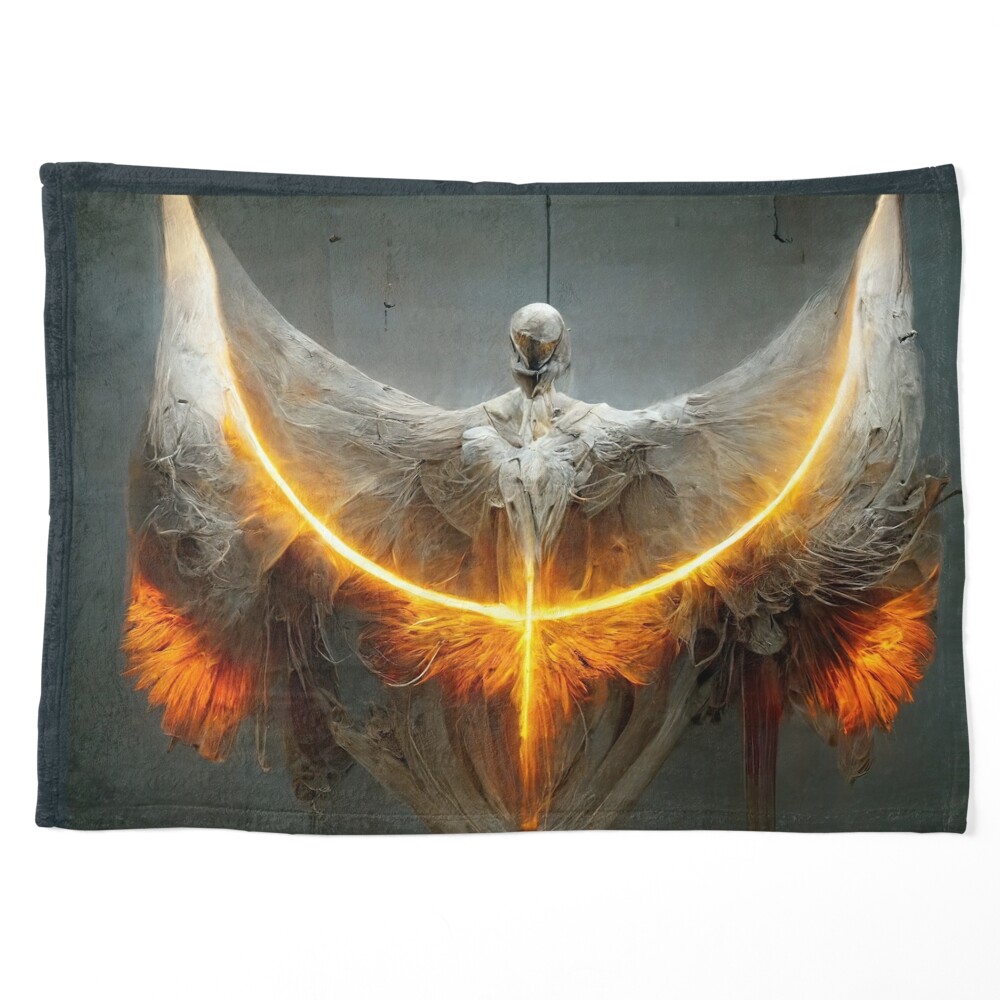The image displays a detailed graphic reminiscent of a set of angelic wings outstretched on a gray to dark gray fabric background, almost like a flag. The wings span from one side to the other, appearing light gray or white with a distinctive cobweb-like texture. A prominent element is a golden-orange line resembling fire, which swoops in a half-moon shape from one wing's top, down and around, finally reaching the other wing. This fiery line also crosses the wings vertically in a T-shape, creating a striking visual effect. The bottom tips of the wings are accented with the same fiery glow. At the center of the wings is a round, glass-like feature, adding to the ethereal nature of the image. This combination of textures and fiery accents against the varying shades of gray fabric creates a dramatic and otherworldly representation.